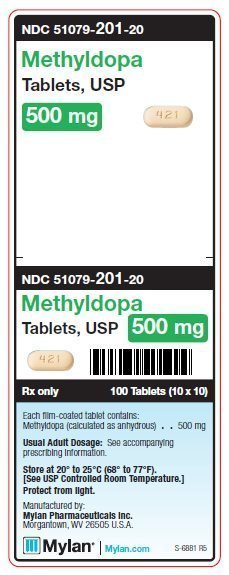**Detailed Caption for the Medicine Label Image:**

In the image, we see the back label of a medicine bottle. At the top of the label, there is a black bar with white lettering displaying "NDC 51079-201-20". Below, the medicine is identified as "Methyldopa Tablets, USP, 500 mg". A visual of the medication is provided, depicting a long, white pill marked with "A21".

Further down, the label reiterates the NDC number, the medicine name, and the dosage. Another picture of the pill is displayed alongside a barcode. The text "RX only" and "100 tablets (10 x 10)" appears next.

On a light blue section of the label, detailed information is listed: "Each film-coated tablet contains methyldopa, calculated as anhydrous 500 mg." The typical adult dosage is provided, with a note to refer to accompanying prescription information. Storage instructions advise keeping the medication at 20°C to 25°C (68°F to 78°F), following USP controlled room temperature guidelines, and to protect it from light.

The manufacturer details include "Mylan Pharmaceuticals Inc., Morganville, WV 26505 USA". A blue and white Mylan logo is shown, with "Mylan" in black letters on a white background, and "mylan.com" underlined in blue. The bottom right of the label features the code "S-6881 FS".